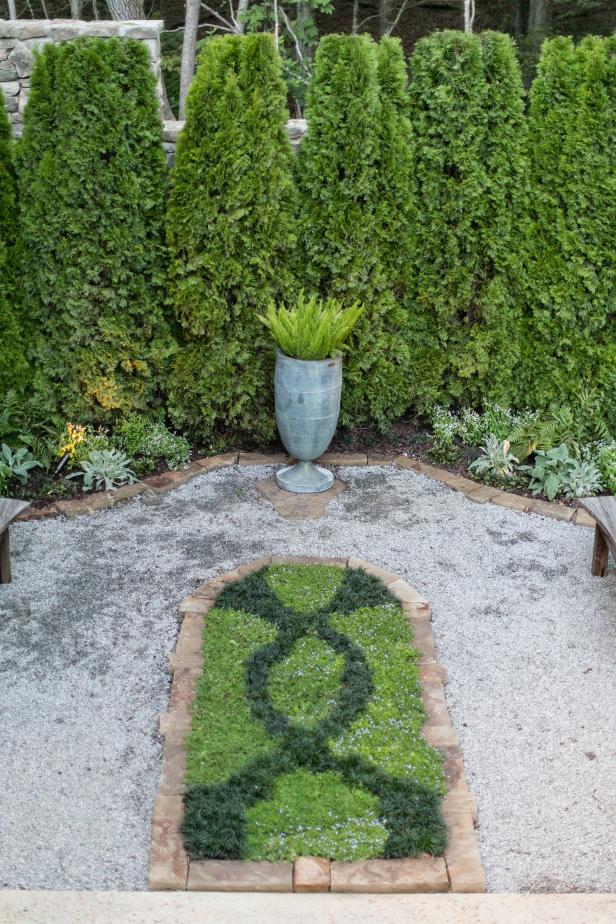The photograph, taken outdoors in daylight using portrait mode, showcases a meticulously trimmed hedge composed of approximately five cone-shaped bushes. These bushes feature a unique form, being broader at the top and tapering slightly towards the bottom, allowing for visible gaps between their peaks. The hedge encircles a cement area bordered with light brown bricks, adding a structured element to the scene. At the bottom of the image, an arch shape made from bricks frames a striking latticework design of two contrasting shades of green plants. Additionally, a silver planter in the background houses vibrant, fern-like plants, contributing a pop of bright green to the composition.